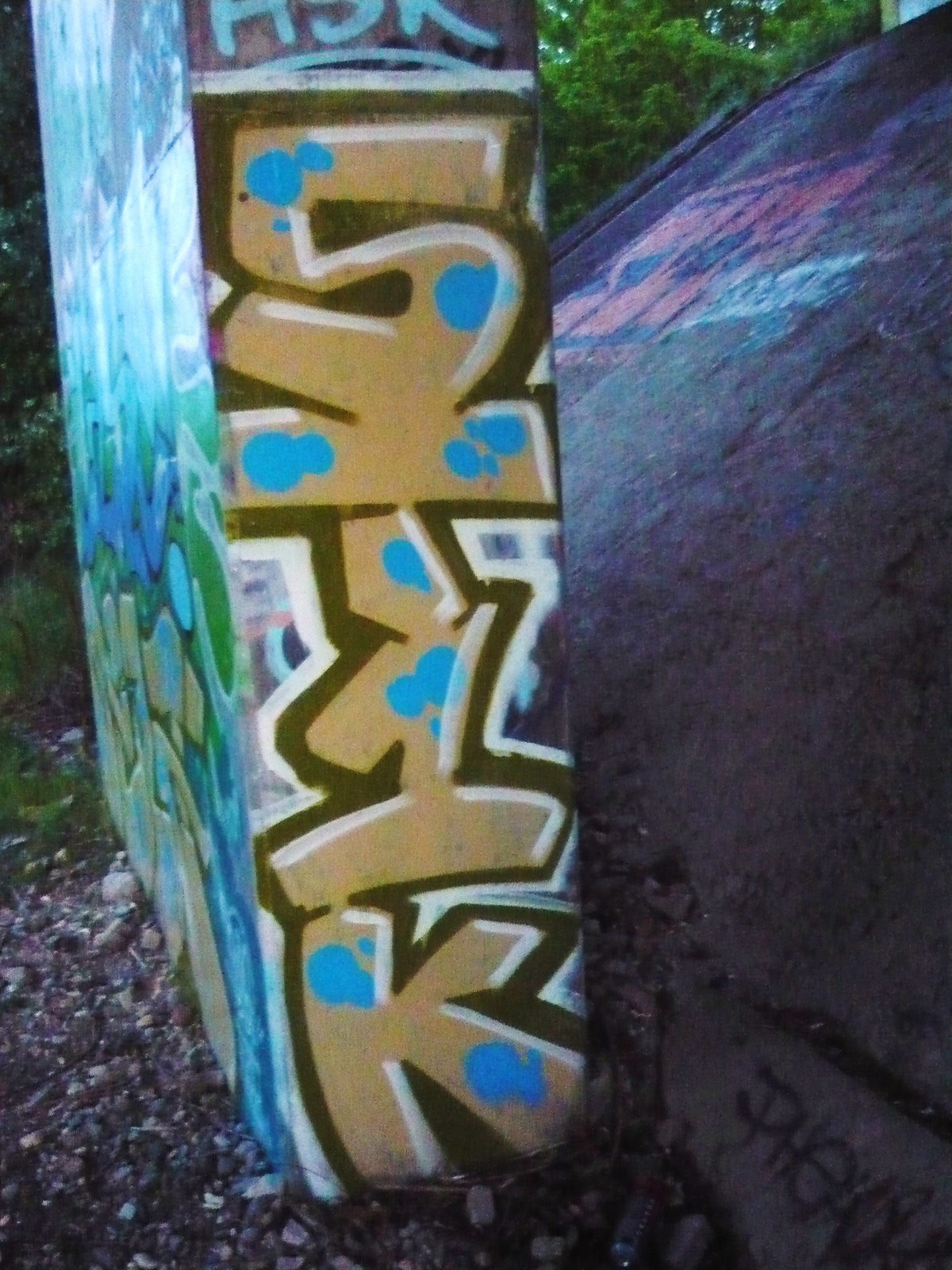This outdoor image captures a scene dominated by vibrant graffiti on a vertical concrete structure, likely a part of a bridge leg or a similar support. The focal point of the graffiti features large, vertical block letters in yellow paint spelling out "5 T 1 K," accentuated with a black drop shadow, white highlights, and blue speckles. Surrounding the graffiti-covered structure, lush green foliage from trees and bushes provides a stark contrast to the urban art. The ground beneath is strewn with small stones and rocks, giving a rugged texture to the area. Adjacent to this structure is another concrete piece, possibly a ramp, further adorned with various colored graffiti, including hues of blue, green, yellow, and purple. The daylight enhances the vividness of the colors, bringing a dynamic sense to the scene. The setting appears to be in a wooded area, park, or possibly beneath a bridge, enhanced by the natural elements and man-made art intermingling.